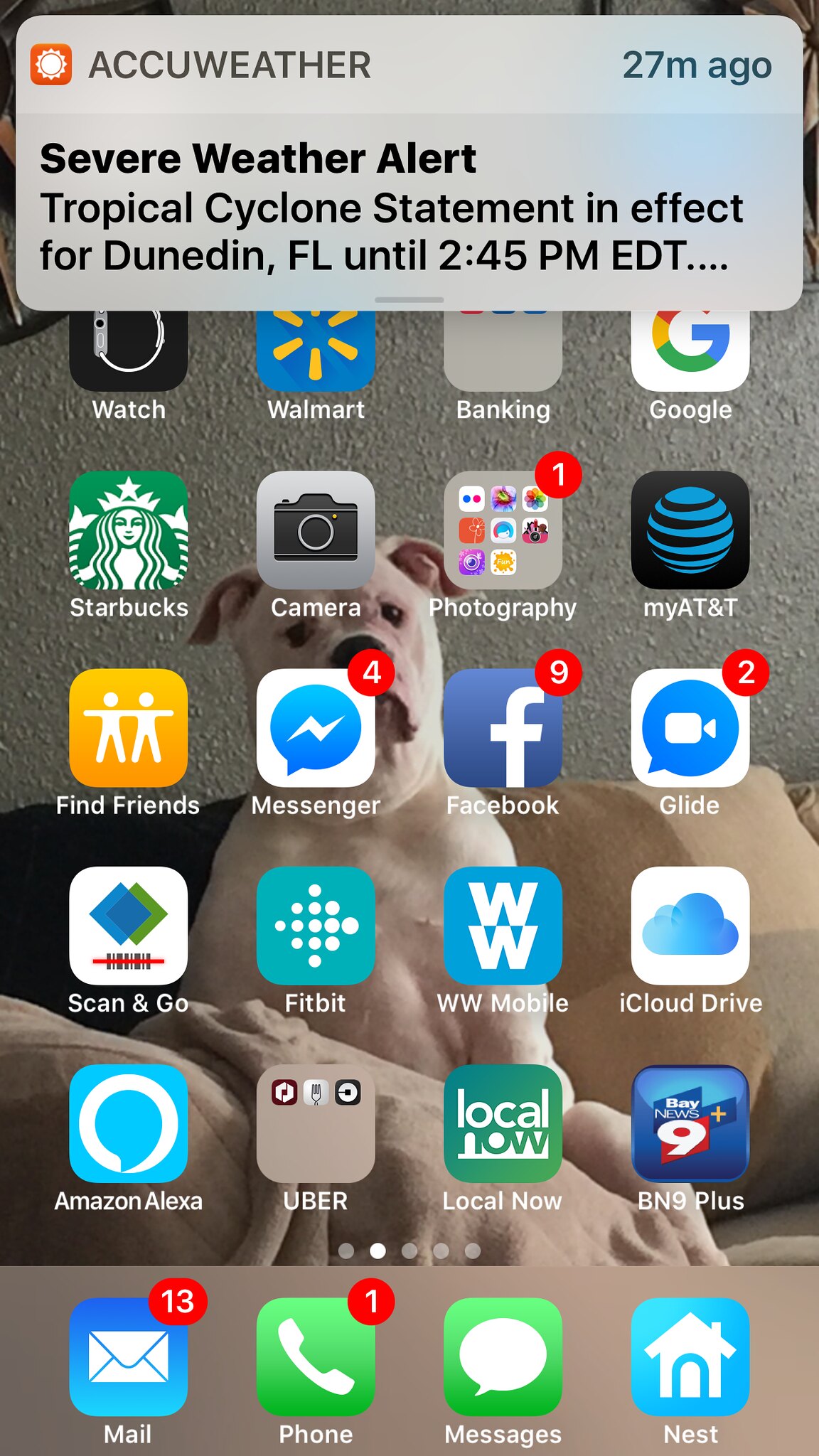A detailed screenshot captured from an iPhone smartphone showcases a weather alert prominently at the top. The alert is from AccuWeather, displayed within an orange box marked by a white sun icon, and was issued 27 minutes ago. The alert banner indicates a severe weather warning, specifically a tropical cyclone statement, in effect for Dundon, Florida, until 2:45 PM EDT.

Beneath the weather alert, the iPhone’s home screen is visible, featuring a wallpaper backdrop of a white bulldog sitting on a black and white couch against a white painted wall. The home screen contains a neatly organized array of apps, with four apps per row spanning a total of five rows. Visible apps include Starbucks, Camera, myAT&T, Find Friends, Messenger, Facebook, Fitbit, and Amazon Alexa, among others.